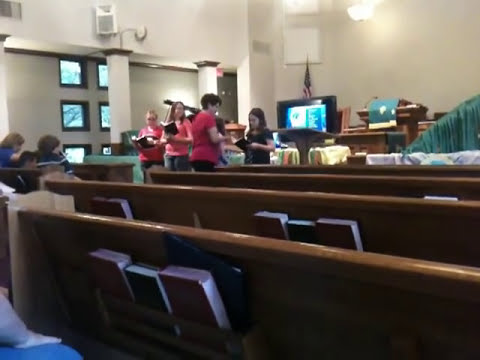Inside a well-lit church with white or cream-colored walls, there is a scene centered around a corner formed by two walls opposite the viewer. In the foreground, several brown pews can be seen, each with books stored on the shelves at the back, likely hymnals or Bibles. To the left side of the photograph, windows allow natural light to pour into the room. At the front of the church, a group of four people, including a woman and what appears to be two children, are engaged either in reading or singing from open books. They are accompanied by another person, making a total of three individuals with books. An American flag is positioned behind the group, and a draped pulpit is also visible. Two additional people are seated in a pew at the far end, participating in this seemingly serene and communal gathering.